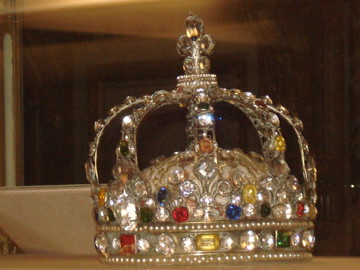This rectangular, low-quality vintage photograph captures an ornate crown displayed indoors, possibly in a museum. The crown is housed in a wooden display case with a glass front and is resting on a white shelf against a brown background. The crown itself is a stunning mixture of gold and silver, adorned with a plethora of jewels in various colors—ruby red, sapphire blue, emerald green, onyx black, topaz yellow, and sparkling white diamonds. The base of the crown features a band of inset gems, including vibrant yellow, gold, red, white, and green stones, as well as a border of opulent white pearls. The rounded top section is encrusted with large jewels and is framed by four gem-studded arms that converge at an intricate, expanded cross-shaped emblem at the peak, which is also decorated with tiny, sparkling diamond-like jewels. The photograph’s quality suggests it was taken with an older camera, giving the image a slightly dated and possibly replica-like appearance.